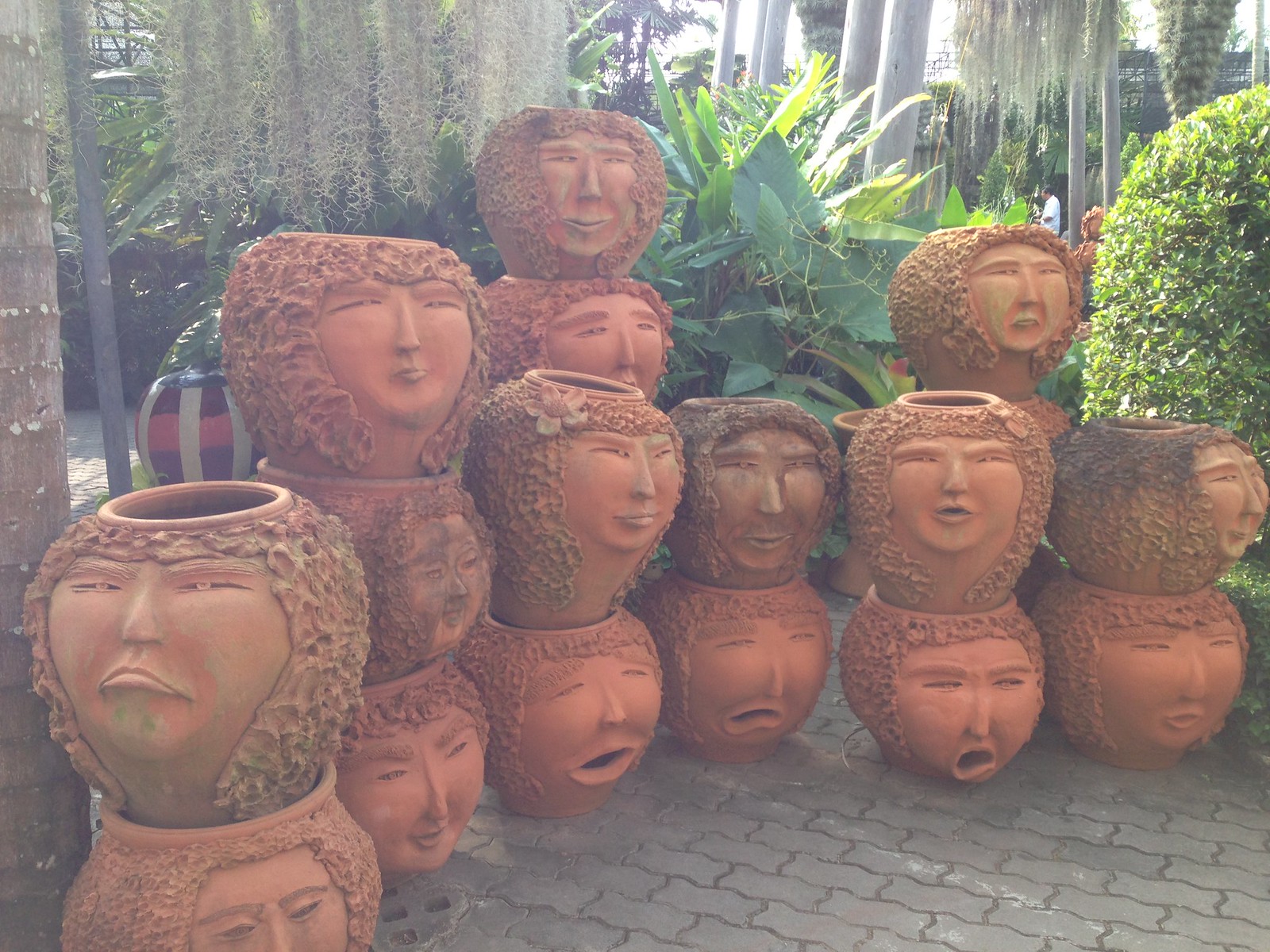In the foreground of the photograph, there is an array of 16 terracotta pots, each meticulously crafted to depict a human face with curly hair carved into the sides. The expressions on the faces are diverse: some smile warmly, others frown, while a few appear to be in distress with mouths agape as if crying. Each pot’s design includes distinct slit-like eyes and holes in the fronts, suggesting a functional as well as artistic purpose. The pots rest on a curvy gray brick surface, and in the background, a lush, jungle-like landscape flourishes with tall, skinny white and tan tree trunks, large green bushes, and spiky plants, including a notable palm-like tree. Among the verdant scenery, there's a man with dark hair dressed in a white T-shirt visible towards the right of the photograph. Overhead, tan, stringy plant elements hang down, adding to the exotic, curated outdoor environment that seems designed for visitors to enjoy.